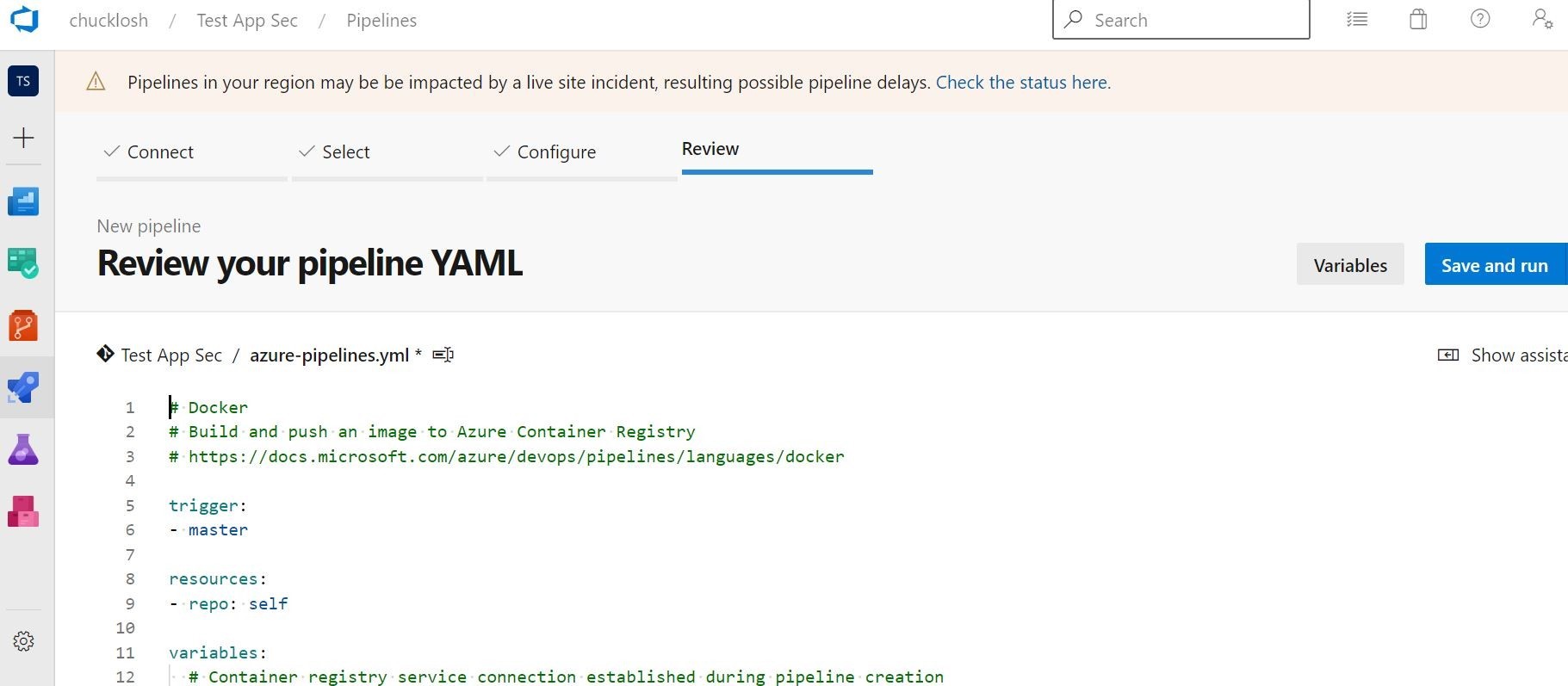The image portrays a detailed review interface, presumably within a Microsoft Office-like environment. The central focus is on a user engaged in reviewing items, with a substantial block of code displayed in the background. A search bar is prominently placed in the top right corner. The interface appears to offer multiple navigational options, including tabs labeled "Connect," "Select," "Configure," and "Review."

Directly below these tabs, there is a section titled "Review Your Pipeline, YAML," with specific references to "Test AppSec, Azure Pipelines, YML" beneath it. On the right side of the interface, options labeled "Variables" and "Save and Run" are visible, suggesting functionality for variable management and execution of tasks.

The left side of the screen features various widgets commonly associated with Microsoft Office Suite applications, contributing to a familiar user experience. Additional details include another search bar and a cluster of symbols at the top right, enhancing the navigability of the interface.

Moreover, an item labeled "Chuck Lodge Test AppSec and Pipelines" is seen on the left side, indicating a specific project or task within the review process. The interface is equipped with a multitude of options and tools, aligned with the user's need to navigate and select tasks efficiently within the Microsoft framework.